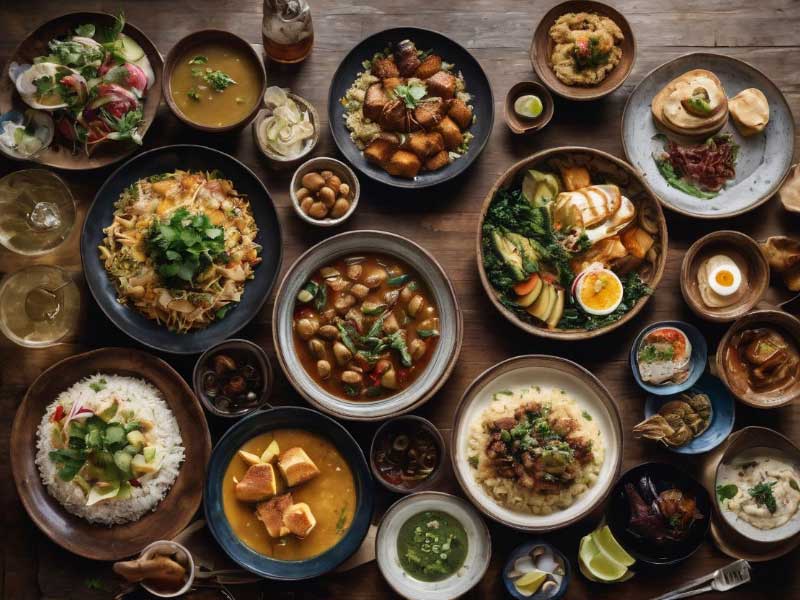This overhead color photograph brilliantly captures a bountiful spread of diverse dishes arranged on a large brown wooden table. The table is adorned with probably a couple dozen plates, varying in colors from brown and black to white, blue, green, and red. The plates themselves range from flat dishes to bowls, each holding a myriad of foods. The array includes rice dishes garnished with pickled cucumbers, pad thai, horseradish, soups with greens, fried bread, and potatoes in a thick sauce topped with basil leaves. There's also a fried rice dish with meat, a salad with pieces of fruit and vegetables, and dishes with beans, limes, eggs, and bagels. Among the utensils, metal tongs are visible on the lower right. To the left, two empty tumblers sit alongside a small glass pitcher filled with an amber liquid in the upper middle. Despite the vast array, the setup is strikingly clean and organized, featuring a mix of circular plates and bowls that lend the table a colorful and vibrant appearance, suggesting a Mediterranean theme with elements like tahuli and parsley. The image exudes an almost perfect, possibly AI-generated quality, highlighting a meticulously detailed and vibrant feast.